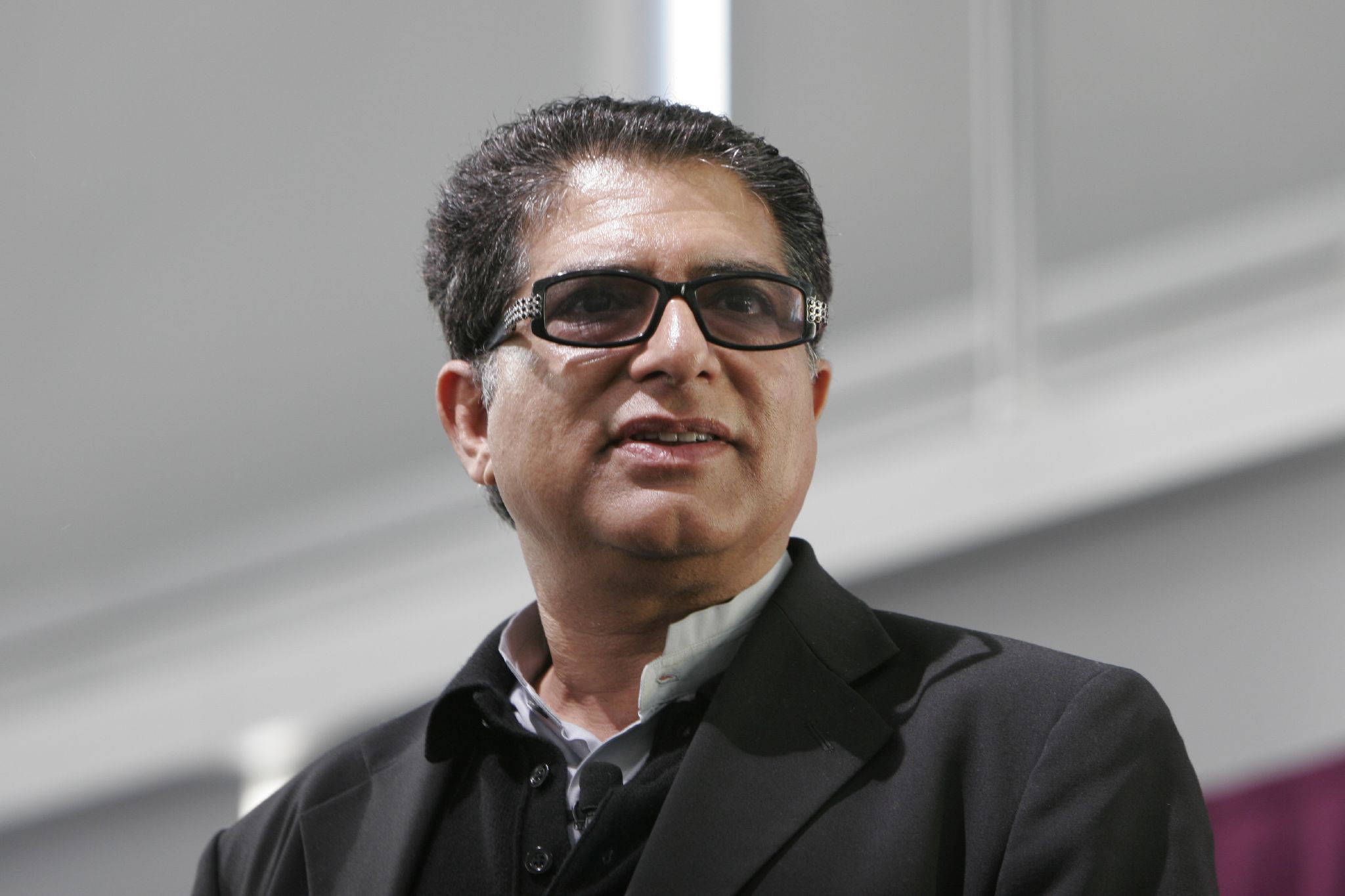In this image, we see a middle-aged man of potentially Indian or Latina descent, situated in the center of the frame. He is wearing dark, black-framed glasses with a silver and black pattern along the stems, which appear to be transition lenses currently dimmed by light. His dark hair is cut short and styled up and back, likely with some product. He is dressed in a black suit and a dark shirt layered over a white button-up shirt.

The man is looking slightly to his right with his mouth open, suggesting he may be speaking or reacting to something off-camera. The background, rendered in bokeh, is slightly blurred but gives an impression of an indoor setting during the day. There is a maroon or burgundy-colored banner or curtain in the lower right part of the image and the rest of the backdrop consists of off-white, white, and tan hues, indicating a possibly institutional or conference room environment. No text is visible in the image.